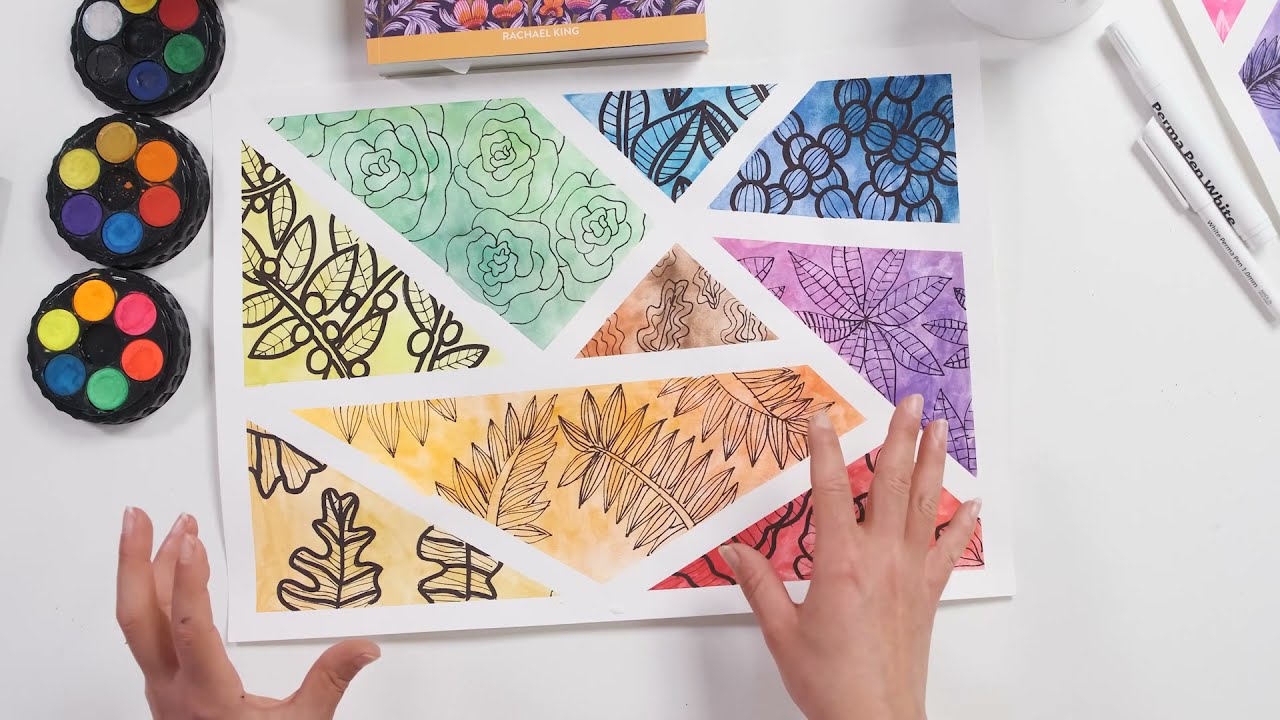The image captures a detailed scene of an artist immersed in their creative process. The centerpiece features a watercolor artwork segregated into nine distinct geometric sections, each vividly colored with hues ranging from yellow and orange to green, blue, purple, red, and brown. Black-painted foliage patterns adorn each segment, lending a bold contrast to the vibrant backgrounds. Surrounding the artwork, on a pristine white table, three circular palettes containing an array of paints are positioned to the left, each palette holding six different colors. The artist’s hands, slightly tanned and free of nail polish, hover near the bottom of the frame above the painting, poised as if ready to continue working. In the upper right of the image, various art supplies including pens, a white marker, and a book with a purple and red cover titled "Rachel King" with gold trimming, are partially visible, suggesting a comprehensive creative setup. The scene is meticulously arranged, emphasizing both the intricate artwork and the tools of the trade.